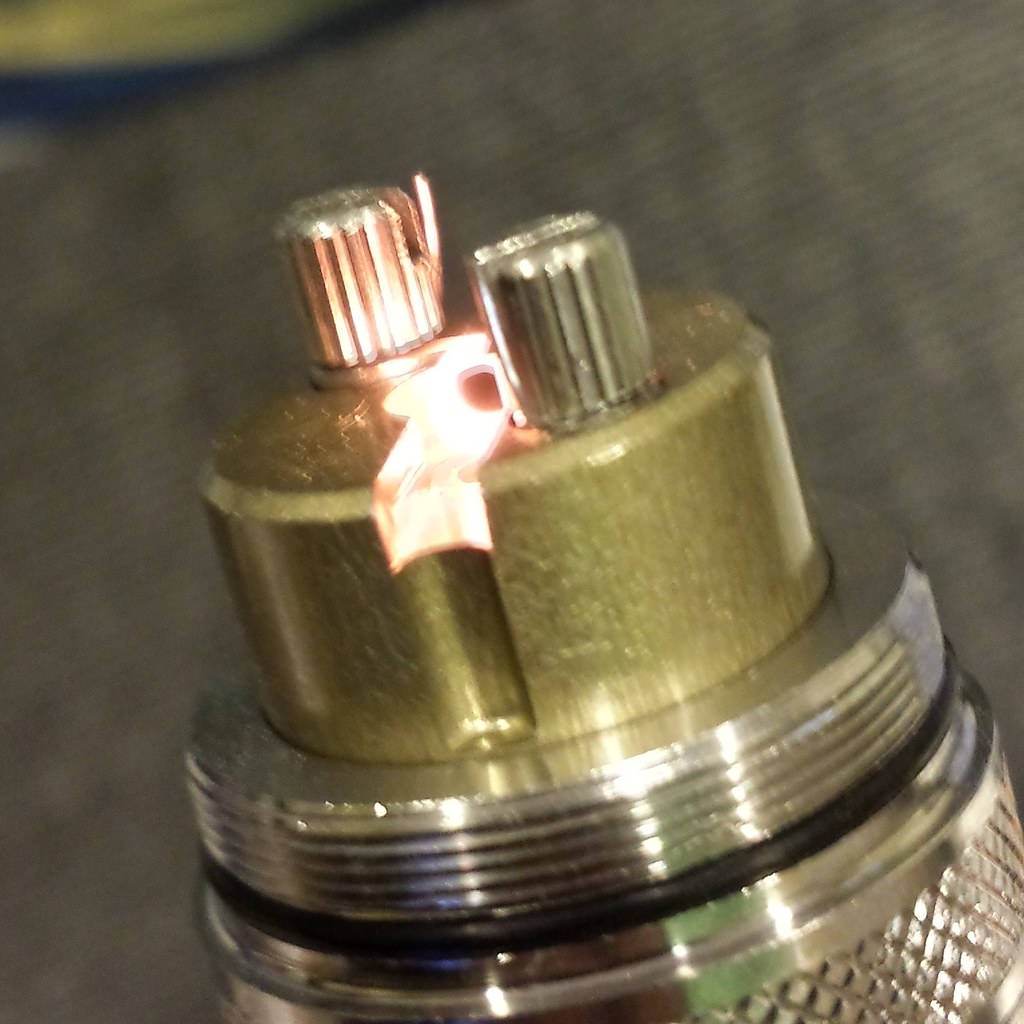This is a detailed close-up photograph of a cylindrical, metal tool that dominates the center of the image, extending diagonally from the bottom right corner. The primary material appears to be silver, with an intricate diamond pattern at the bottom right section, followed by a screw-on design and a black rubber ring encircling this part. Above the black ring, the tool features a smaller, gold-colored cylindrical section. The very top of the tool comprises two side-by-side cylindrical prongs with flathead screwdriver slots, between which a subtle orange hue is reflected, likely due to light striking the object. The background is a dark grayish-brown fabric, adding contrast and causing some reflections on the tool. The overall image is slightly blurry, with light glancing off the top and sides, highlighting the metallic components.